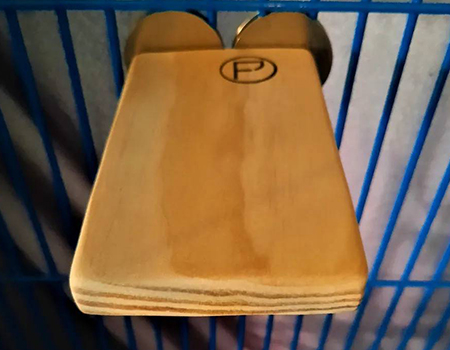The image showcases a striking blue gate constructed from vertically arranged, heavy wire bars. About three-quarters of the way down, these bars are intersected by a horizontal bar, all uniformly painted in a deep blue color. In the center of the gate, near the top, two reflective, golden discs are prominently welded. Extending out from these discs is a smoothly sanded, light brown wooden plank, approximately two inches thick, projecting perpendicularly toward the camera. Notably, to the top left of the wooden plank, there's an engraved dark circle with the letter "P" inside it, possibly a brand mark. The overall composition suggests a unique, possibly improvised structure, with a backdrop hinting at a concrete wall behind the blue railing. The interplay between the bright blue bars, golden discs, and the engraved wooden plank creates a visually intriguing and detailed scene.